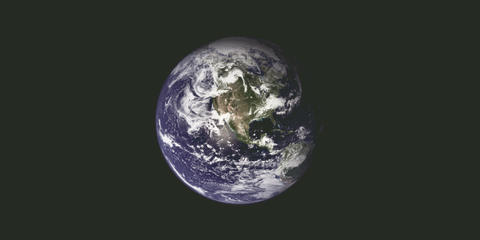This image showcases the planet Earth from a great distance, likely taken from space or high orbit. Earth is situated in the center of the image and contrasts starkly against a completely black background, emphasizing the isolation of our planet in the vastness of space. The photograph reveals a detailed view of the Earth's land masses and vast oceans. North America is particularly discernible, along with hints of Middle and South America. The land is a patchwork of greens and browns, while the oceans are rendered in varying deep shades of blue. Scattered across the globe are white, wispy clouds, swirling around and partly obscuring the surface, indicating weather patterns. The depiction of Earth is simple yet evocative, capturing the spherical shape and the dynamic, ever-changing atmosphere of our planet, making it a stunning representation of Earth as seen from space.